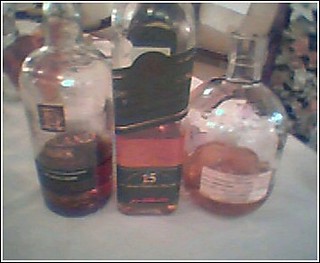This blurry, older, and low-quality color photograph captures three partially emptied liquor bottles resting side-by-side on a white surface. Each bottle contains a dark amber liquid, suggesting they hold scotch or whiskey. 

The bottle on the left is rounded with a black label that has gold lettering near the bottom. Its contents are mostly depleted, showcasing a clear, reddish liquid. Additionally, a hint of a possibly 'R' shaped logo can be faintly seen. 

The taller, more squared bottle in the middle also features an illegible black and gold label, and holds a dark liquid, with its level also significantly reduced. 

The bottle on the right is the shortest and has a jug-like shape with a white label. Unlike the other two, it appears to lack a cap and what remains inside is ambiguous, perhaps indicating the presence of some residue. 

Overall, the photograph’s poor focus and small size make finer details hard to discern, but the distinguishing shapes and labels of each bottle are still apparent.